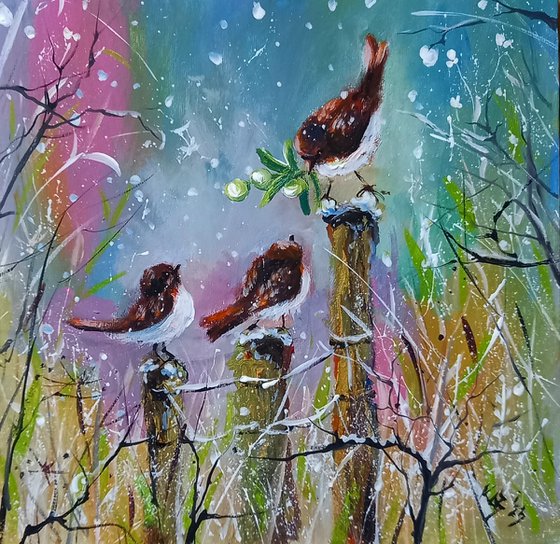The painting depicts a trio of vibrant red cardinal birds, each with striking white underbellies, perched on individual fence posts. The central bird stands prominently on the middle post, with another bird on a slightly higher post to its left, suggesting a familial arrangement. Below them, the posts are painted in a yellowish-brown hue. The background captivates with its gradient of colors, transitioning from pink on the left to shades of blue, white, and green on the right, enhanced by streaks throughout. Tree limbs, dark brown and black, adorned with white speckles indicative of snow, frame the scene at the base. This harmonious blend of vivid wildlife and dynamic color palette renders the painting a beautiful and evocative winter landscape.